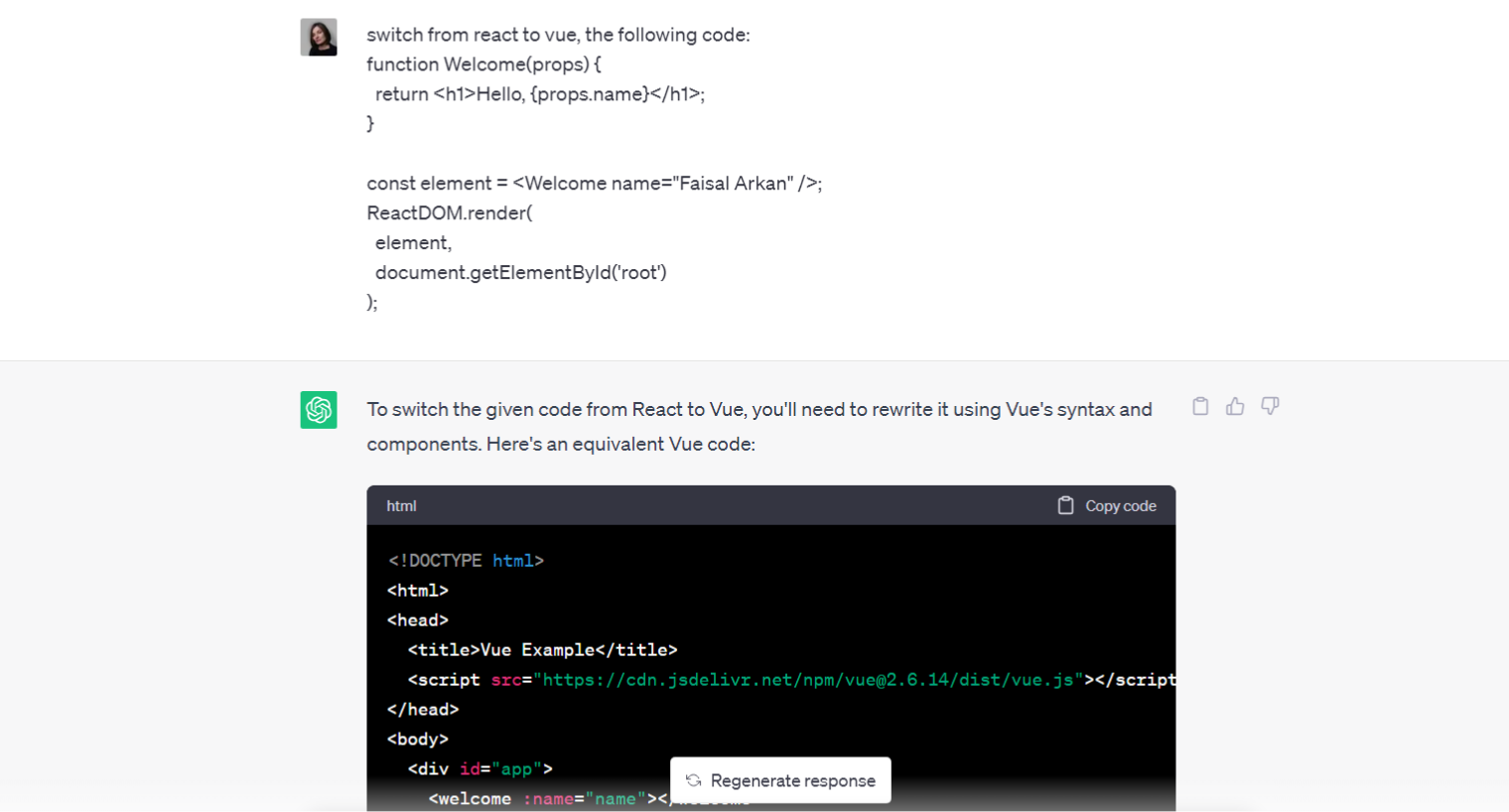The image displays a series of coding instructions, beginning with a depiction of a person inside a gray box to the left. To the right of this visual, text guides the user on switching from React to Vue (spelled V-U-E). The detailed instructions start with:

```
function welcome(props) {
  return <h1>Hello, {props.name}</h1>;
}
```

Following this, there's an additional section introduced after a blank space:

```
const element = <Welcome name="FAISALARKAN" />;
ReactDOM.render(element, document.getElementById('root'));
```

Next to this, another gray box features a green symbol, resembling a rose flower, with a message indicating that to transition the provided code from React to Vue, one must use Vue's syntax and components. Below this message, a black box contains the Vue equivalent code. Within this layout, a white box is prominently displayed, labeled "Regenerate response."